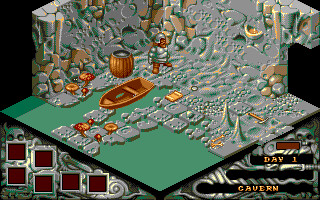The small, detailed image appears to be a screen capture from a video game, depicting a cavern scene. The picture features a green and silver color palette set against a black background. At the bottom, there is green water, above which spreads a path of grey stones leading to a grey shore. Within this scene, notable elements include a boat, a barrel, and a humanoid figure with brown skin, white hair, and a white tunic. 

In the lower left-hand corner, there are six silver rectangles with red squares in the middle, aligned within a white pattern. The left side of the image features a greenish pattern against a black background, with the words "Day 1" and "Cavern" written in gold or copper. These words appear in the lower portion of the screen. This intricate arrangement of graphical elements suggests the image is part of a schematic representation within the cavern setting of a video game.